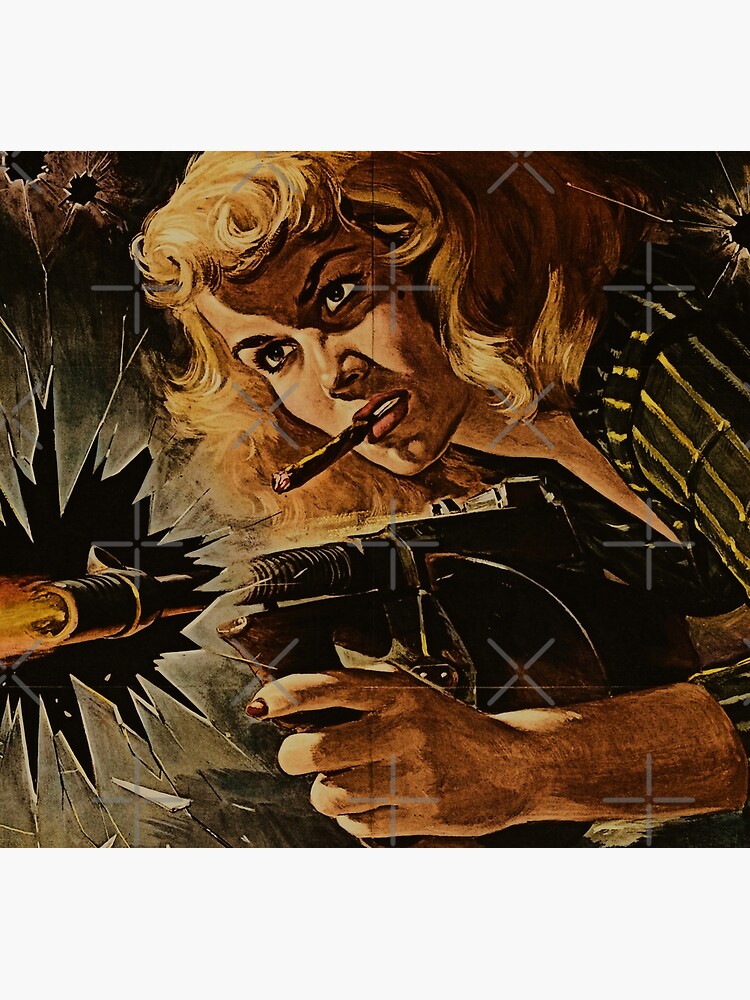The image depicts a stylized, cartoonized illustration of a blonde woman with wavy, curly hair and bangs, intensely focused as she fires a tommy gun. She is hunched over to the left, seen from the right side, gripping the foregrip of the gun with her left hand, her painted red fingernails visible. A cigar or cigarette clenched between her teeth adds to her fierce expression, with her dark brown arched eyebrows highlighting her determination. She is dressed in a pinstriped black and white shirt, reminiscent of a gangster’s suit. The flash of the tommy gun is stylized with black and orange colors, with cracks emanating from it, and two bullet holes are visible against the brown, abstract background. Shards of glass fly, suggesting she shot through a window, with the vibrant scene framed in various shades of yellows, tans, golds, blacks, and grays. Subtle water markings in the form of a cross add an artistic touch to the composition.